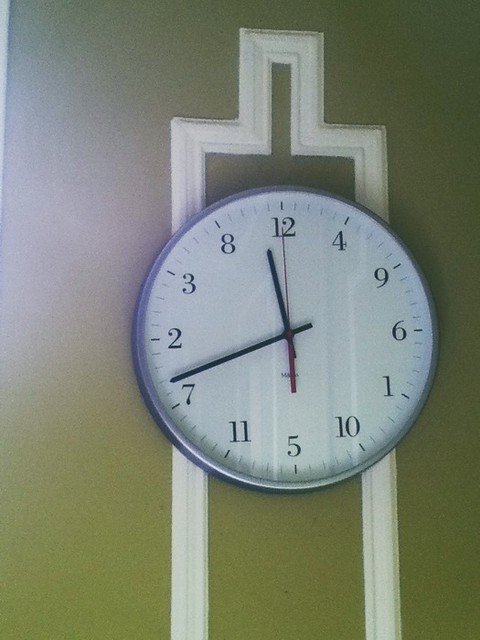This image depicts a unique wall clock. The clock has a round face with numerals placed in an unconventional order. Starting at the top center with the number 12, the sequence continues clockwise with 4, 9, 6, 1, 10, 5, 11, 7, 2, 3, 8, and back to 12. The clock features three different hands – a short black hand indicating the hour, a longer black hand signifying the minutes, and a slender red hand for the seconds. The wall behind the clock is a greenish color, and there is a distinct white rectangular design in the background, adding an additional element of interest to the overall visual composition.